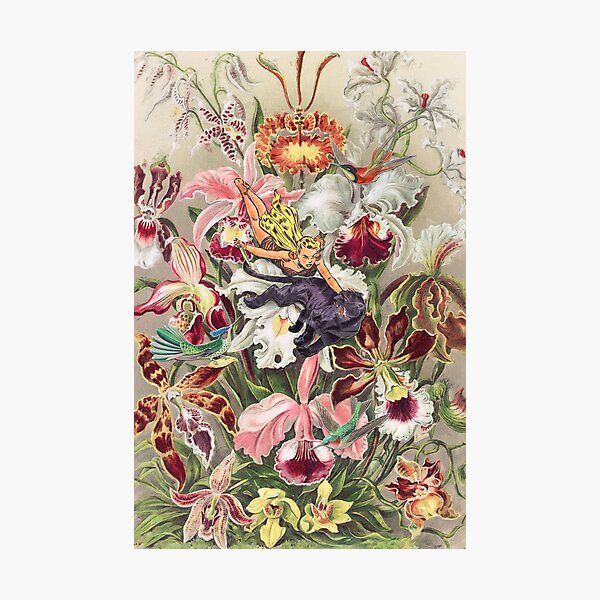The image is a detailed, vintage botanical painting with an antique feel, showcasing a large collection of exotic flowers against an off-white, cream background. The flowers, which include orchids, snapdragons, lilies, irises, and possibly other varieties, are vividly colored in shades of pink, white, red, orange, yellow, purple, and light green, with lush greenery forming a backdrop. In the midst of this floral abundance is a diminutive fairy, depicted with yellow wings and blonde hair, appearing to fly down towards the flowers. Notably, the scene also features a dramatic encounter between a woman adorned in a brown tiger-striped dress, and a jaguar. The woman, who has flowing blonde hair, is grasping the jaguar's neck with one hand while wielding a dagger in the other. A small hummingbird rests on a flower petal, seemingly observing the intense interaction. The intricate blend of the fairy, the combat, and the vibrant flora creates a captivating and surreal visual experience.